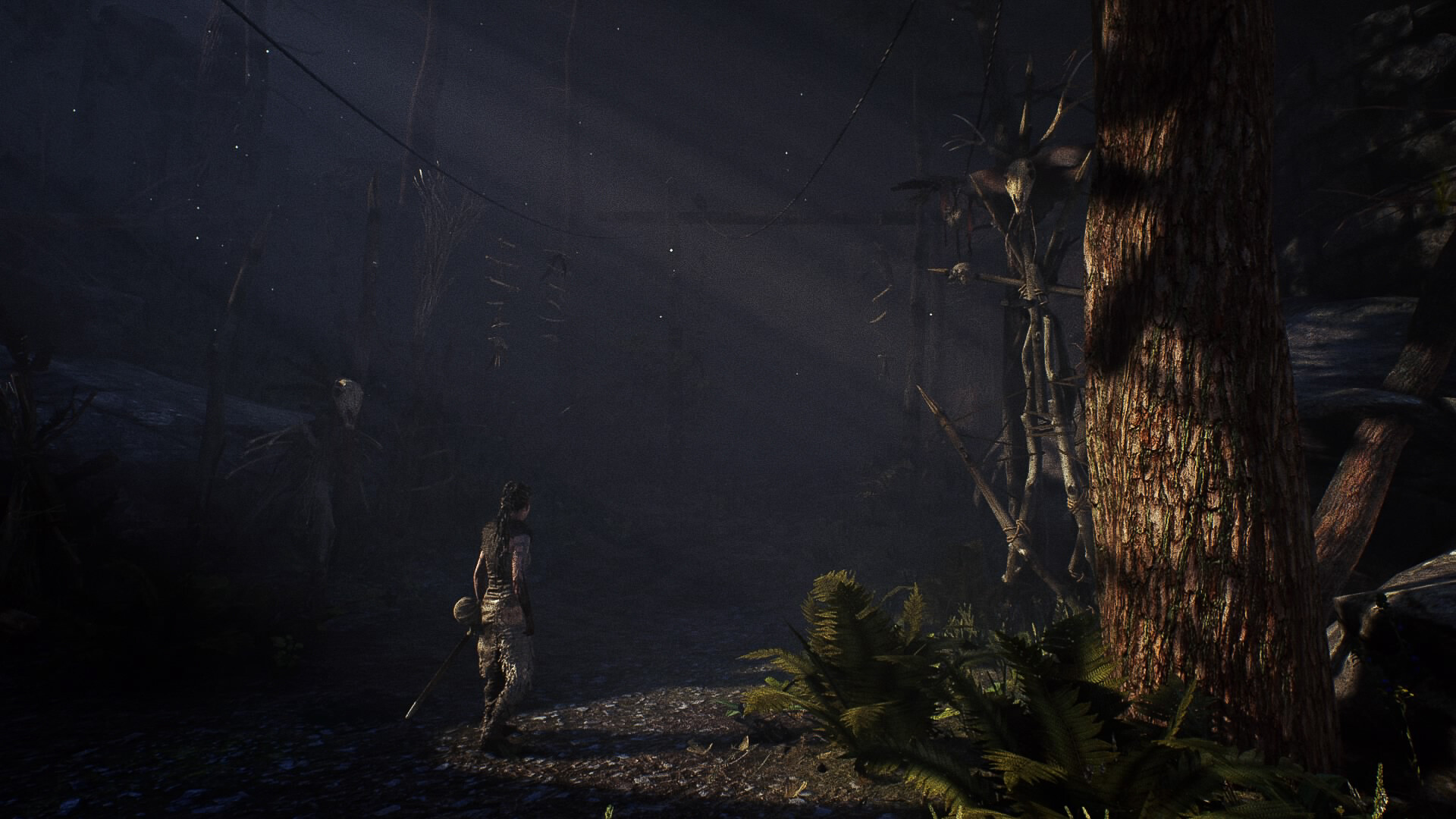In this nocturnal screenshot of a video game, a character navigates through a dense forest. Dominating the right side of the scene is a colossal tree, its base adorned with lush ferns. To the left-middle of the image, a woman dressed in white pants stands with her back to the viewer, gripping a sword and heading towards the right. Hovering ominously on the left side of the tree, a formidable stick-like monster with a diamond-shaped face and an exaggerated collar behind its head appears to be floating. The creature's spindly body and legs are clearly visible, and it seems to be holding an object near the bottom of its foot. In the murky background, a web of dark wires and indistinct structures adds to the eerie ambiance of the forest at night.